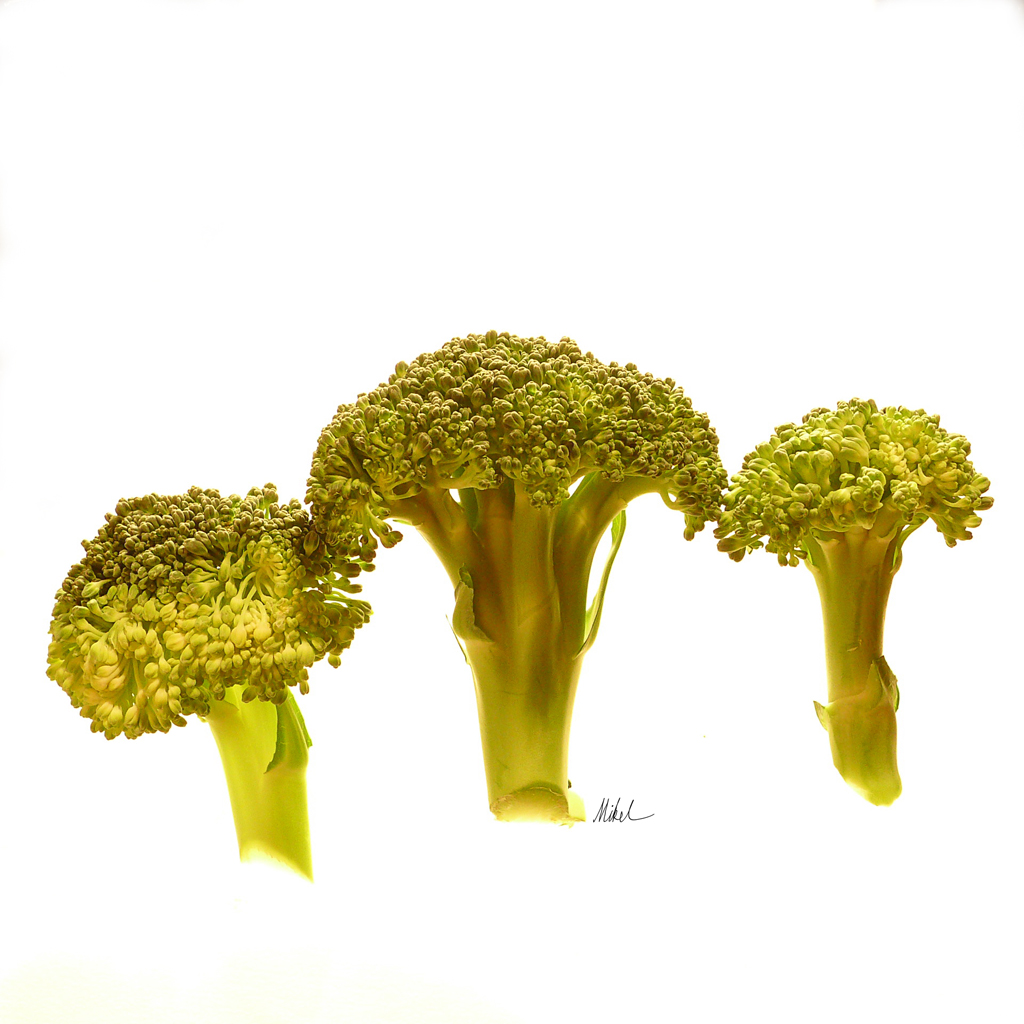This is a detailed depiction of a drawing or photorealistic image of three pieces of broccoli against a white background. The broccoli appears to be somewhat aged or cooked, displaying an unusual color palette that diverges from the typical vibrant green. The central piece of broccoli is the largest, transitioning from a lime green at the bottom to a medium green at the top, with its florets resembling brain matter. To the left, a smaller piece shows a gradation from lime green at the bottom to a darker green at the top, with a yellowish tint in between. On the right, a broccoli stalk taller than the one on the left but shorter than the one in the middle, exhibits medium green hues. The image is signed by the artist, with the signature "M-I-K-E-L" in black penmanship situated near the central stalk. While the authenticity of the broccoli being fresh or cooked is ambiguous, the depiction gives an impression of a drawing intended to capture an unusual and artistic representation of the vegetable.